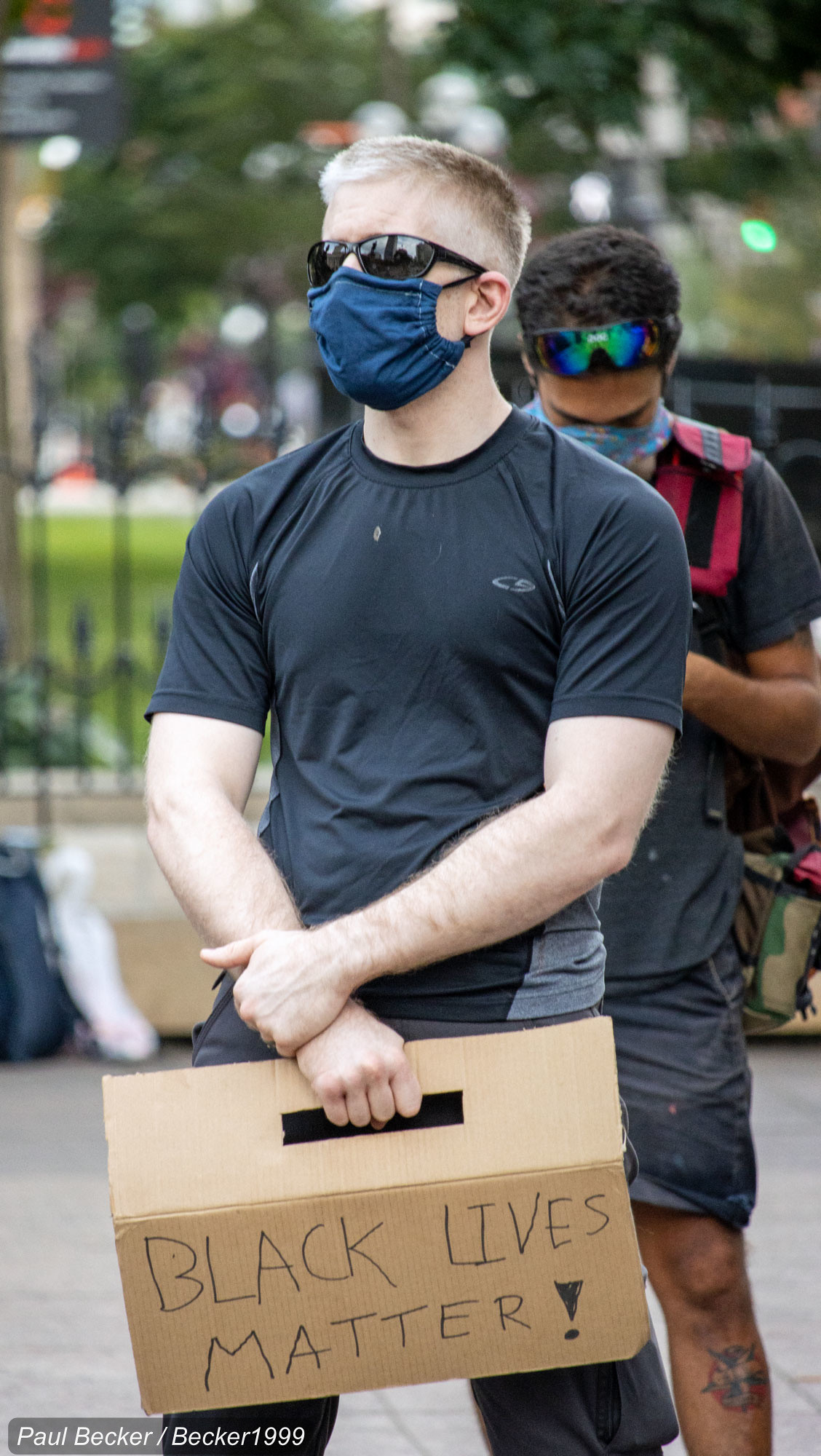The photograph captures a scene from a Black Lives Matter protest, prominently featuring a white man standing in the foreground. He has blonde hair and is dressed in a dark blue shirt, dark shorts, and a blue surgical mask, indicative of the COVID period. He sports dark sunglasses and stands with his arms crossed, possibly focused on a speaker addressing the crowd. In his hand, he holds a piece of cardboard with a handle cut into the side; the visible text reads "Black Lives Matter!" Exclamation Point.

Behind him stands a black man with sunglasses positioned on his forehead and also wearing a mask. A visible tattoo decorates his right leg. The scene is set in a public space, with a metal fence, some grass, and possibly trees and a building in the distance. The ground is scattered with bags, likely belonging to other attendees. The image is credited to Paul Becker, with a watermark reading "Paul Becker/Becker 1999" in the bottom left corner.